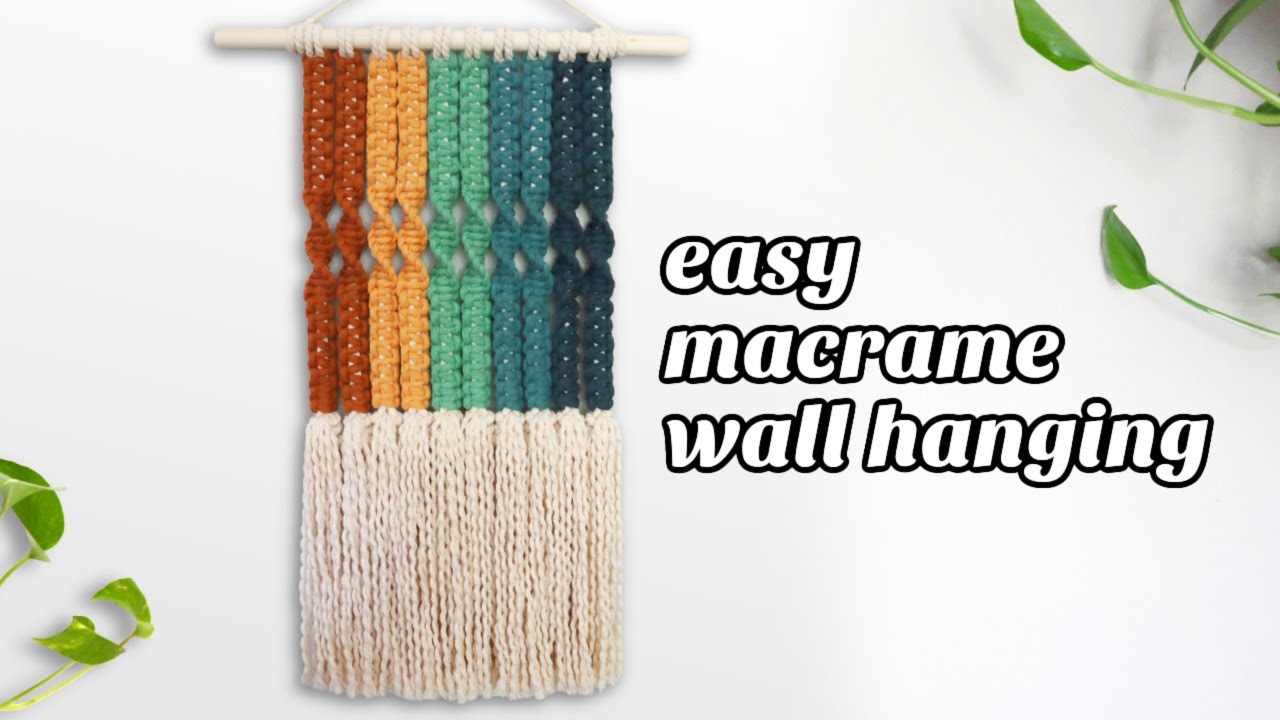The photograph showcases a vibrant macrame wall hanging against a stark white background, likely part of an advertisement. Positioned prominently on the left center of the image, the wall hanging is suspended from a wooden rod and features pairs of tassels in various colors—two red, two orange, two light green, two light blue, and two dark blue—intertwining with a cascade of white tassels descending below. Subtle botanical elements with green leaves peek in from the top right and bottom left corners, adding a touch of nature. To the right of the macrame, the bold white text reads "Easy Macrame Wall Hanging" in a clear, attention-grabbing font. The overall aesthetic suggests a clean, instructional presentation possibly inspired by a YouTube video or a detailed advertisement.